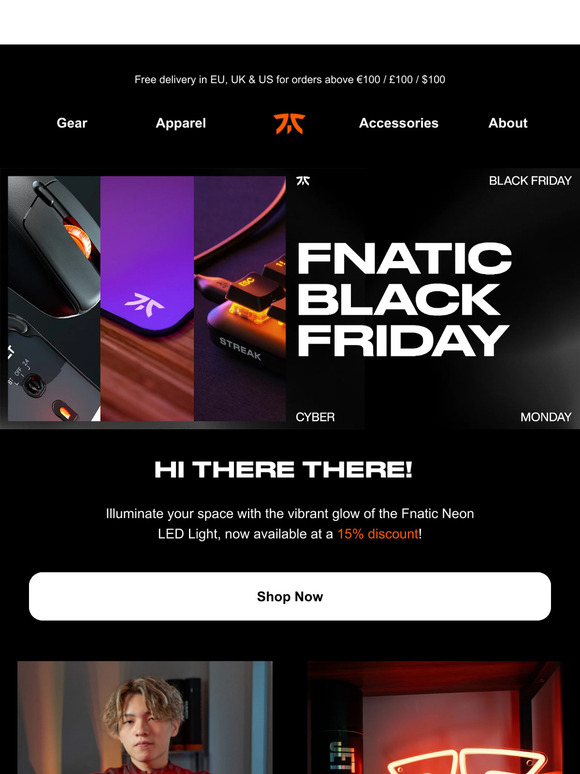A screenshot of the Fanatic shopping website is displayed, featuring a sleek, flat black background. At the top, the logo, a stylized orange design resembling a curvy number seven mirrored with a small orange comma in between, accompanied by the brand name “Fanatic” spelled as “F-N-A-T-I-C,” is prominently shown. Just above, white text announces free delivery in the EU, UK, and US for orders over $100, and also mentions 100 pounds and 100 euros.

Below the logo, the navigation menu options are listed: Gear, Apparel, Accessories, and About. A large banner dominates the center, highlighting a Black Friday sale with Cyber Monday included, featuring a partially visible light-up mouse, the corner of a laptop, and a glowing gaming keyboard against the dark background. On the right side of the banner, bold white text reads, "Fanatic Black Friday and Cyber Monday."

Further down, the text "Hi There There. Illuminate your space with a vibrant glow of the Fanatic neon LED light, now available at a 15% discount," appears. "15% discount" is highlighted in orange, contrasting with the surrounding white text. Beneath this text, a prominent white rectangular button with rounded corners and black text invites users to "Shop Now."

In the lower left corner, there is an image of an Asian man with medium-length blonde hair, which falls just below his ears. Though the exact product he's associated with isn't clear, a light-up neon sign appears on the right side of the section.